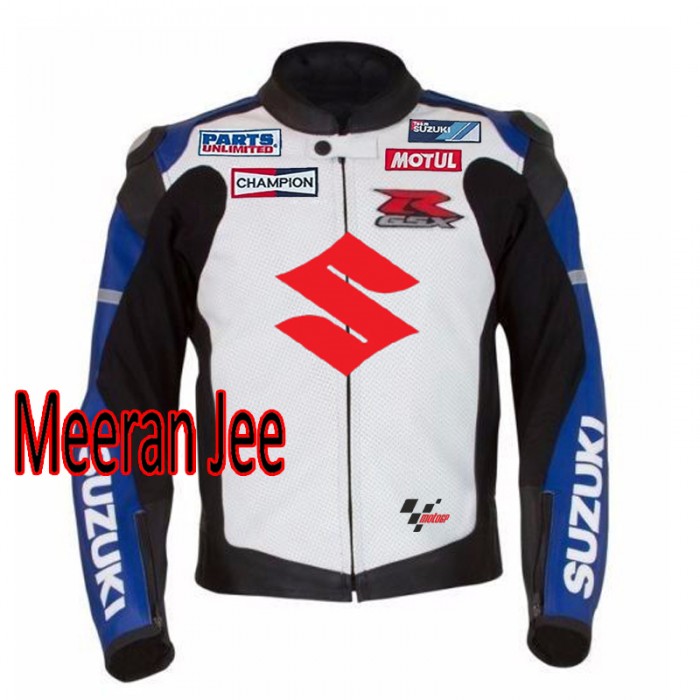This is a professionally taken, color photograph of a Suzuki racing jacket, set against a stark white background that enhances the details of the garment. The jacket features a striking design with a predominantly white chest, black trim, and a large, red Suzuki 'S' logo centered on the front. The collar is black, and the chest area includes several rectangular sponsor patches. Notably, the left chest has a "Parts Unlimited" patch with 'Parts' in blue font and 'Unlimited' in red, and a "Champion" patch featuring black text on a white background. The right chest showcases a "Motul" patch in white font on a red background, a "Suzuki" patch with black, blue, and white diagonal stripes, and a "GSX" logo in gray underneath a red 'R'. 'Suzuki' is displayed in white on the blue portions of both sleeves, which also feature black underarm sections and a distinctive gray band running horizontally on the upper arms. On the bottom left of the jacket, black text with a red outline spells out "Miran GJE" or similar. The jacket's zipper is black, complemented by a white tab at the collar, secured with a black snap, adding both function and a touch of design elegance.